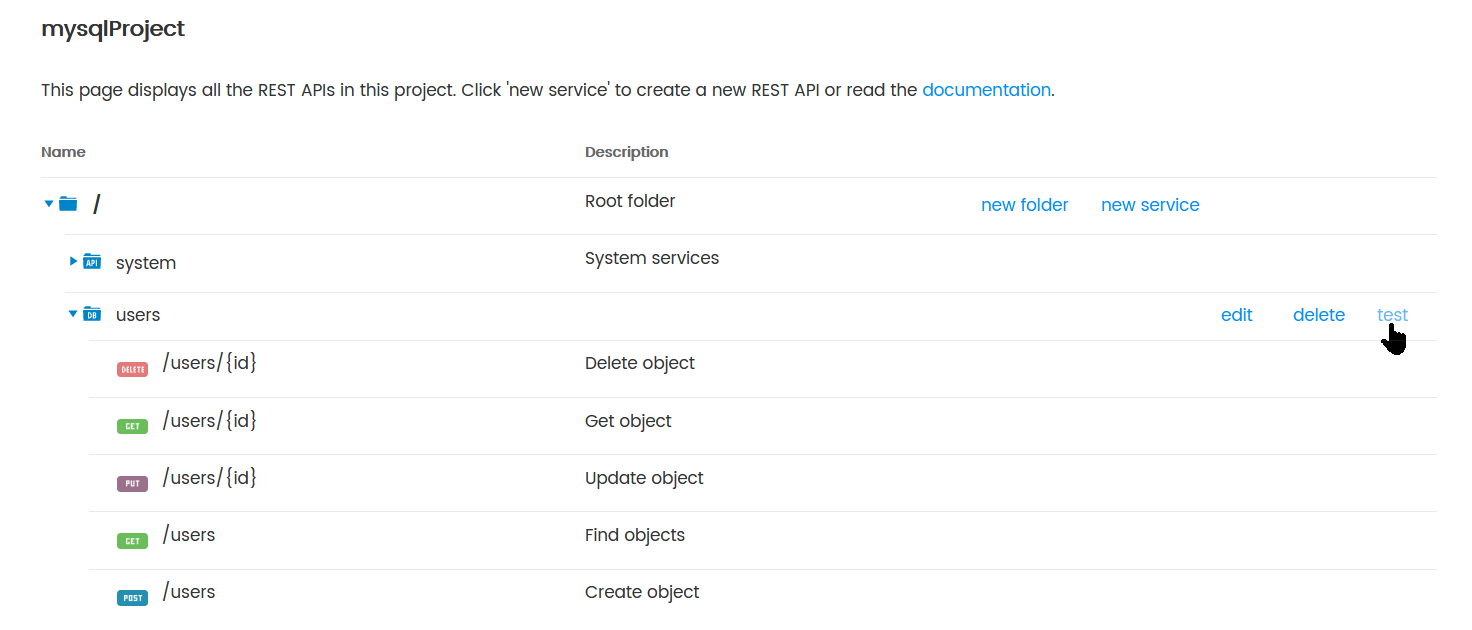The image depicts a digital interface resembling a web-based platform, specifically a SQL project management dashboard. At the top of the interface, a header prominently reads "My SQL Project." Beneath this header, an informative line states, "This page displays all the REST APIs in this project. Click 'new service' to create a new REST API or read the documentation."

The main section of the interface is divided into two primary tabs: 'Name' and 'Description.' Under the 'Description' tab, a list of entries is visible, each representing a different API function within the project. The first entry is labeled "Root Folder," followed by others named "System Services," "Delete Object," "Get Object," "Update Object," "Find Objects," and "Create Object."

Adjacent to each of these descriptions, to the right side of the screen, there are action options marked in blue text. These options are "Edit," "Delete," and "Test," allowing users to manage each specific REST API directly from the interface.

The overall design is clean and functional, with the intention of providing users with a straightforward way to view, create, manage, and test REST APIs within their SQL project.